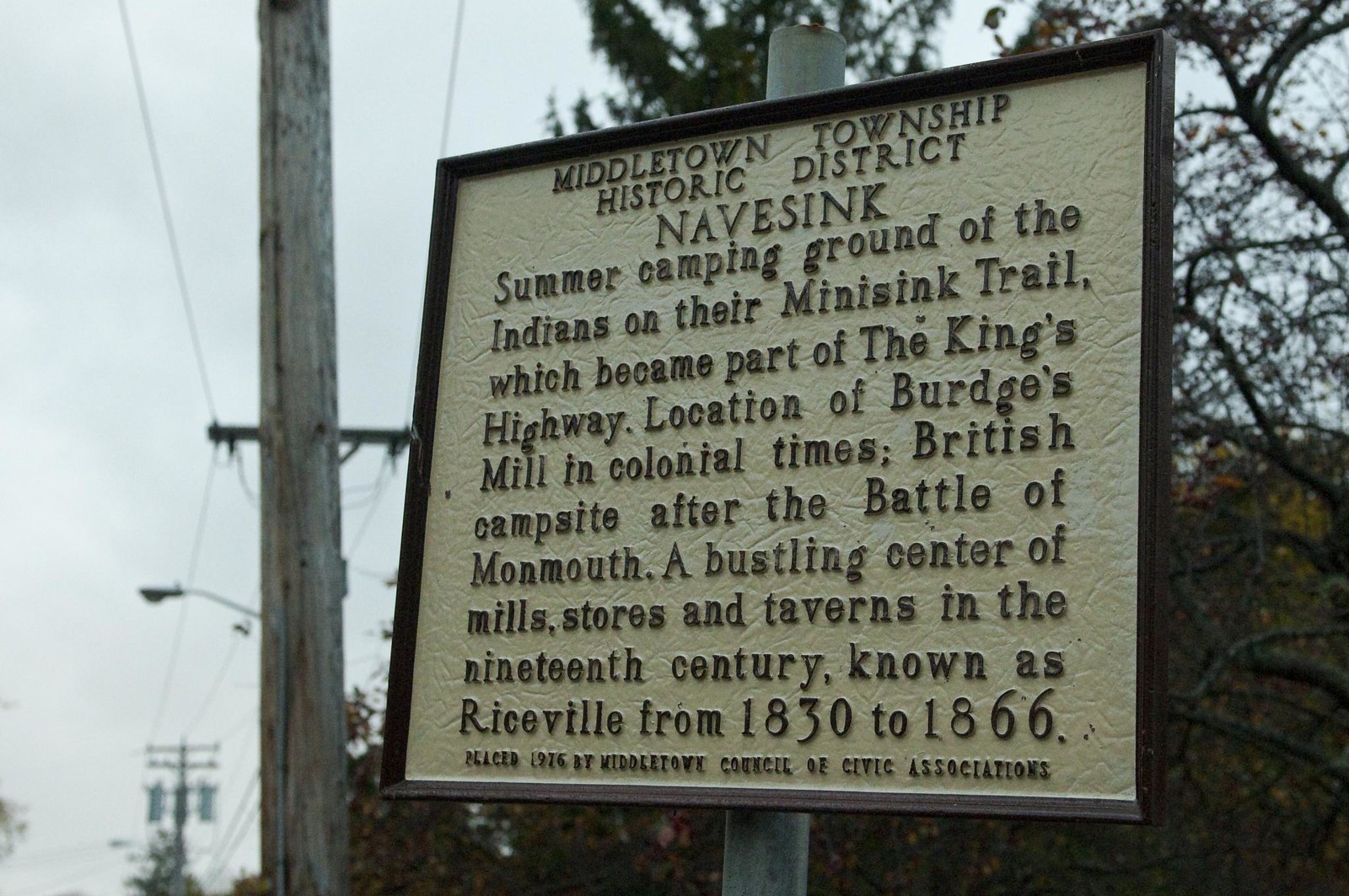The image depicts a scene taken outdoors on an overcast day, under a sky filled with dark clouds. The background includes a mix of leafless trees and electrical poles with wires, suggesting early spring or late fall. In the center foreground stands a metal pole holding a plaque bordered in dark brown with a light tan background. The plaque features dark brown lettering that reads, "Middletown Township Historic District. Navisink, summer camping ground of the Indians on their Minisink Trail, which became part of the King's Highway. Location of Burgess Mill in colonial times. British campsite after the Battle of Monmouth. A bustling center of mills, stores, and taverns in the 19th century known as Riceville from 1830 to 1866." Below the main text, in smaller letters, it says, "Placed 1976 by Middleton Council of Civic Associations." The immediate surroundings suggest a neighborhood setting with a telephone pole to the left and a tree to the right of the plaque.